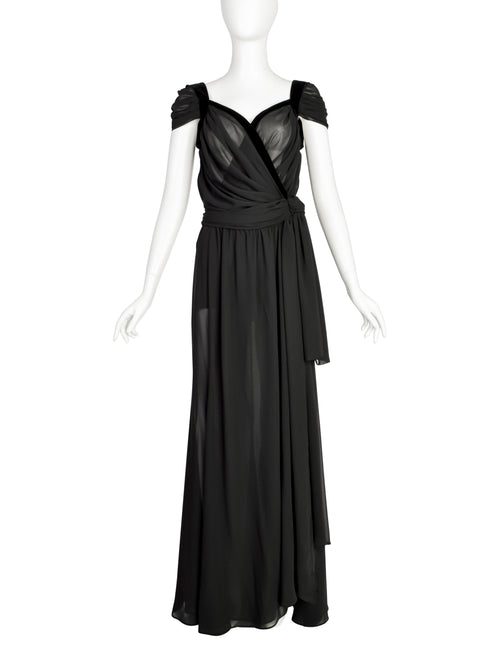The image captures a stark white mannequin donned in an elegant, floor-length black dress designed for formal occasions such as a black-tie wedding. The dress features a sheer, see-through fabric around the chest area, revealing the mannequin's white skin underneath. The dress is meticulously layered, with fabric bunched and draped across the front from both the left and right sides, leading into a sashed black tie cinching at the waist. The dress has very short sleeves and flows gracefully to the ground, fully concealing the mannequin's feet. The mannequin stands with arms positioned by its sides, devoid of facial features, highlighting the dress against a minimalist white background.